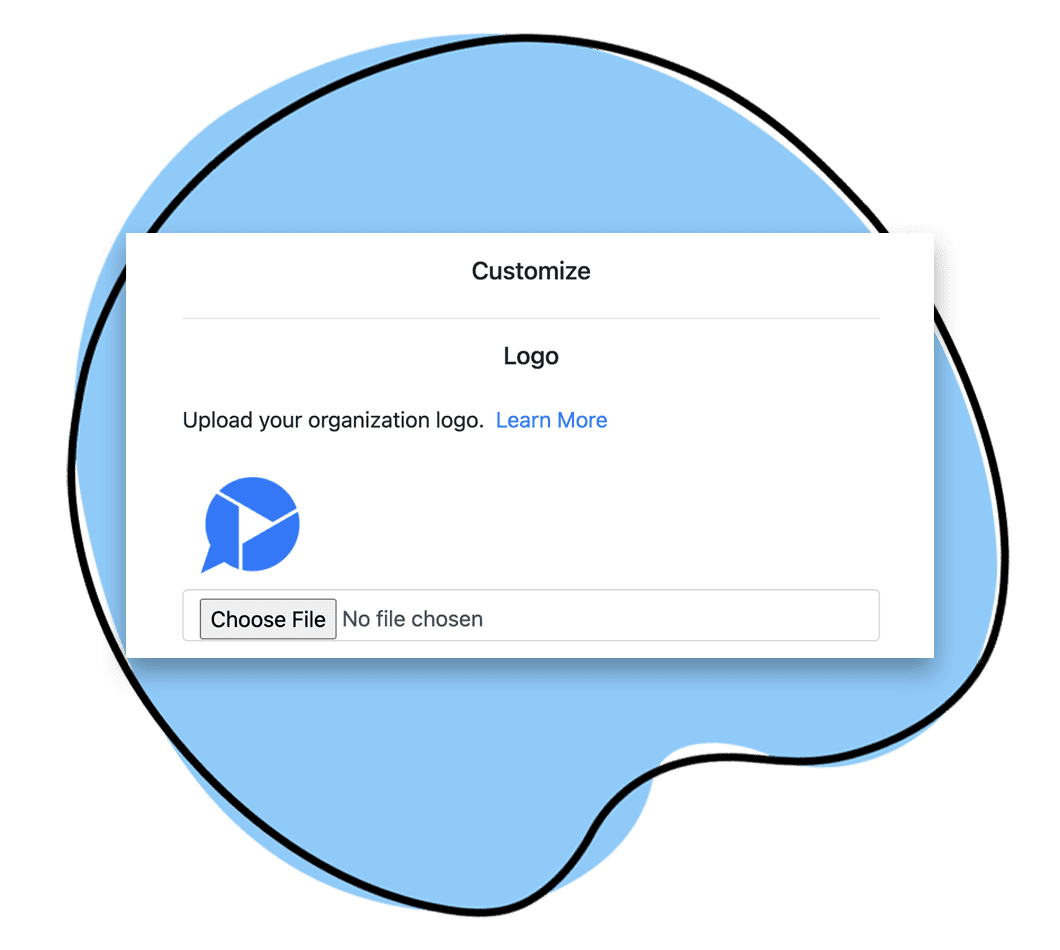This is a screenshot of a pop-up window from a web page, designed for customizing merchandise with an organization’s logo. The pop-up is titled "Customize" and features a section labeled "Logo" with an invitation to "Upload Your Organization Logo." Below this, there is a hyperlink labeled "Learn More" for additional information. In the lower left corner, there is a button labeled "Choose File," which allows the user to select an image file from their computer to upload as their organization’s logo. This logo can then be used to order various types of custom merchandise from the website, such as cups, hats, t-shirts, stationery, office supplies, posters, and even large banners. This is part of an e-commerce platform designed to facilitate the creation and purchase of personalized items for businesses.